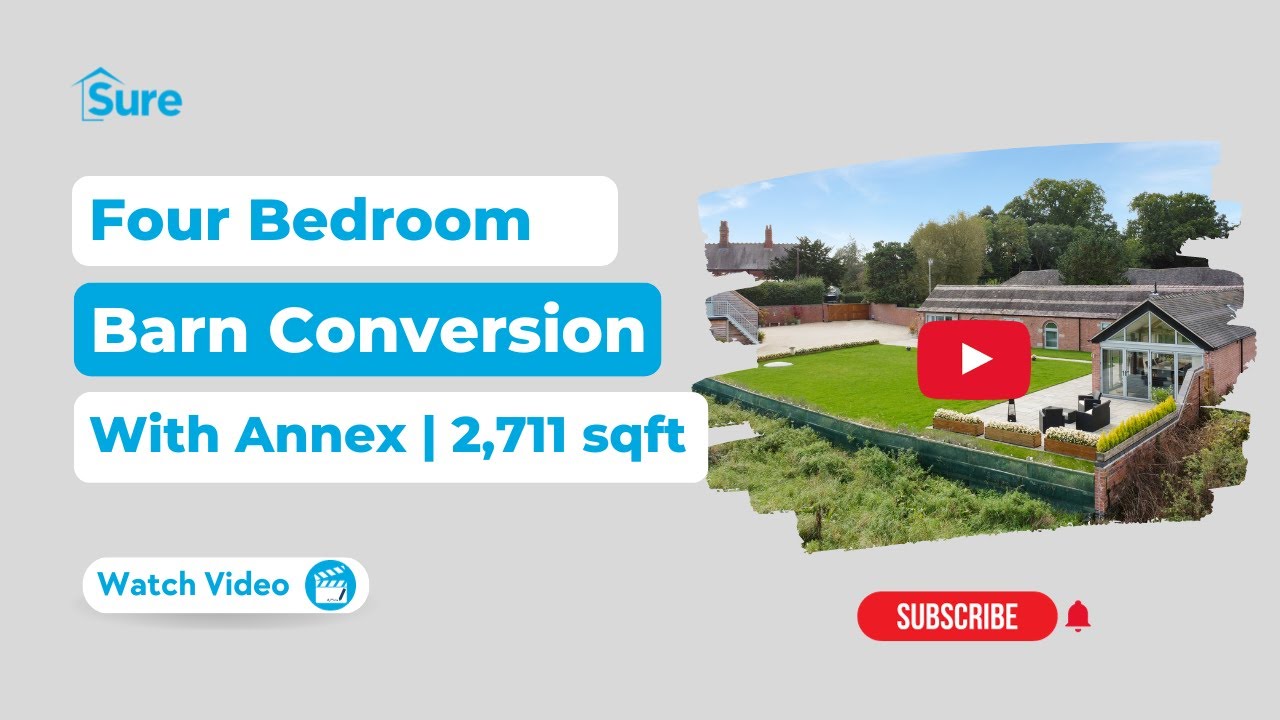This is a title card for a YouTube video showcasing a 4-bedroom barn conversion with an annex, covering 2,711 square feet. The background is light gray. In the top left corner, there is a blue logo with the word "Sure" and an outline of a house around the 'S'. Below this, in a series of blue and white banners, it details the property's type: "4-Bedroom Barn Conversion with Annex," followed by "2711 Square Feet." A "Watch Video" button with a movie clapboard icon is also present. On the right side, there’s a photograph of the property, featuring an L-shaped pink building with a gray roof, a glass-walled end with an outdoor patio seating area, and a bright green lawn with shrubbery. A red YouTube play button overlay signifies that clicking will lead to a video tour. Below this image in a red banner, the white text reads "Subscribe," accompanied by a bell icon for notifications.